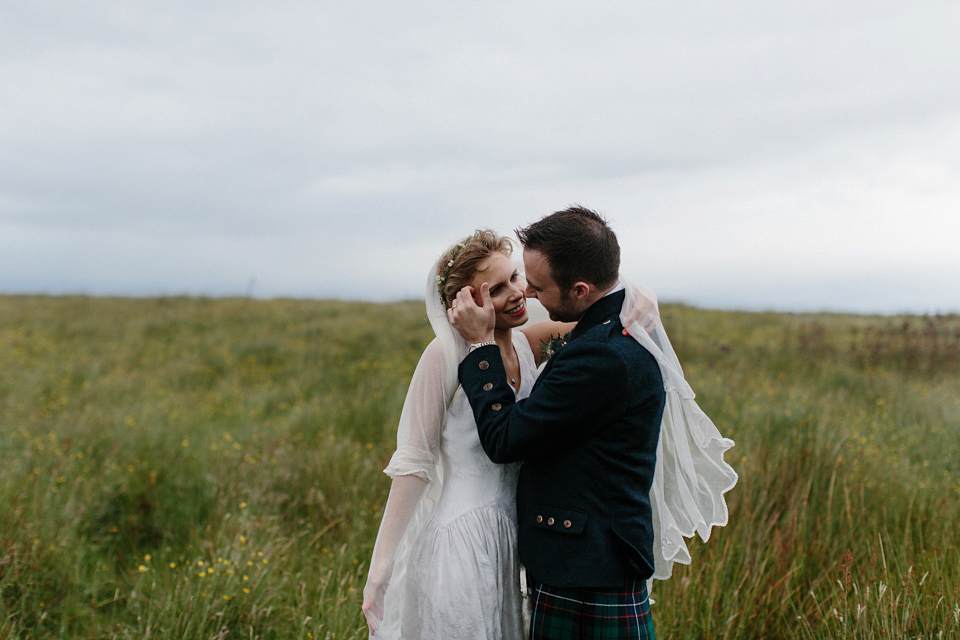In this wedding photoshoot, a newly married couple stands in a picturesque grassland with abundant green vegetation and tall grass, accentuated by small yellow flowers and brown bushes. Overhead, a mostly cloudy sky forms the backdrop with occasional patches of blue. The bride, a fair-skinned woman with light blonde hair styled neatly, wears a flowing white bridal gown with full sleeves and a floral headband. Her left arm lovingly wraps around the groom’s neck, with part of her veil draping over his shoulder. The groom, a fair-skinned man with short brown hair and a beard, is attired in a dark green jacket adorned with golden buttons and a plaid kilt, giving a nod to what seems like a Scottish or Irish theme. He tenderly caresses the bride's face with his left hand as they both smile warmly at each other, encapsulating the joy and intimacy of their special day.